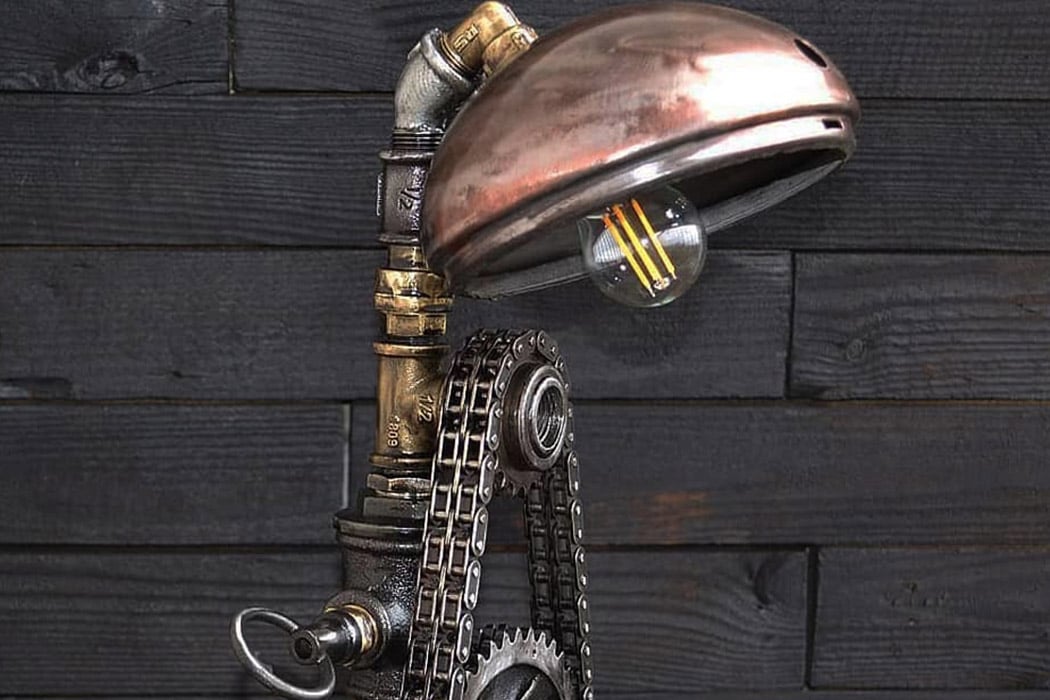The image depicts a steampunk-inspired, mechanized lamp set against a dark grayish-brown, wooden wall. The lamp's design incorporates several intricate elements, including a dome-shaped lampshade that appears to be repurposed from copper metal. A filament-style light bulb with three yellow rods protrudes from the bottom of this lampshade. The lamp features an arched arm constructed from various small pipe fittings. Attached just below the lampshade is a T-section pipe fitting, which supports a small gear with two silver bike chains draped over it. These chains connect to a larger sprocket or gear with teeth. The lamp is adorned with a golden and pewter-colored pin and a metal ring, which add to its mechanical aesthetic. The wall behind the lamp consists of wooden planks with a visible grain, contributing to the overall industrial vibe of the scene.